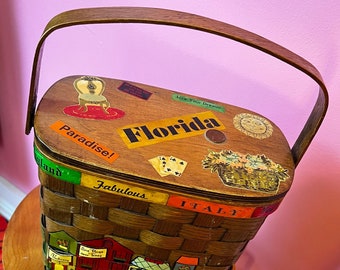The image showcases a medium brown wicker picnic basket with an interwoven pattern of lighter and darker shades. The basket, featuring a sturdy U-shaped handle and a solid wood top, is adorned with an array of colorful decals. Prominently displayed on the lid are a yellow sticker that reads "Fabulous" and an orange sticker that says "Italy." Additionally, there are stickers of playing cards, a Queen's chair, flowers, and the word "paradise" with an exclamation point, among others, making the basket lively and visually engaging. This basket is placed on a light brown wooden circular end table, with a bright pink wall featuring a white border serving as the backdrop. The photo captures the basket from a slight angled perspective, emphasizing the eclectic collection of stickers and the intricate weave of the wicker.